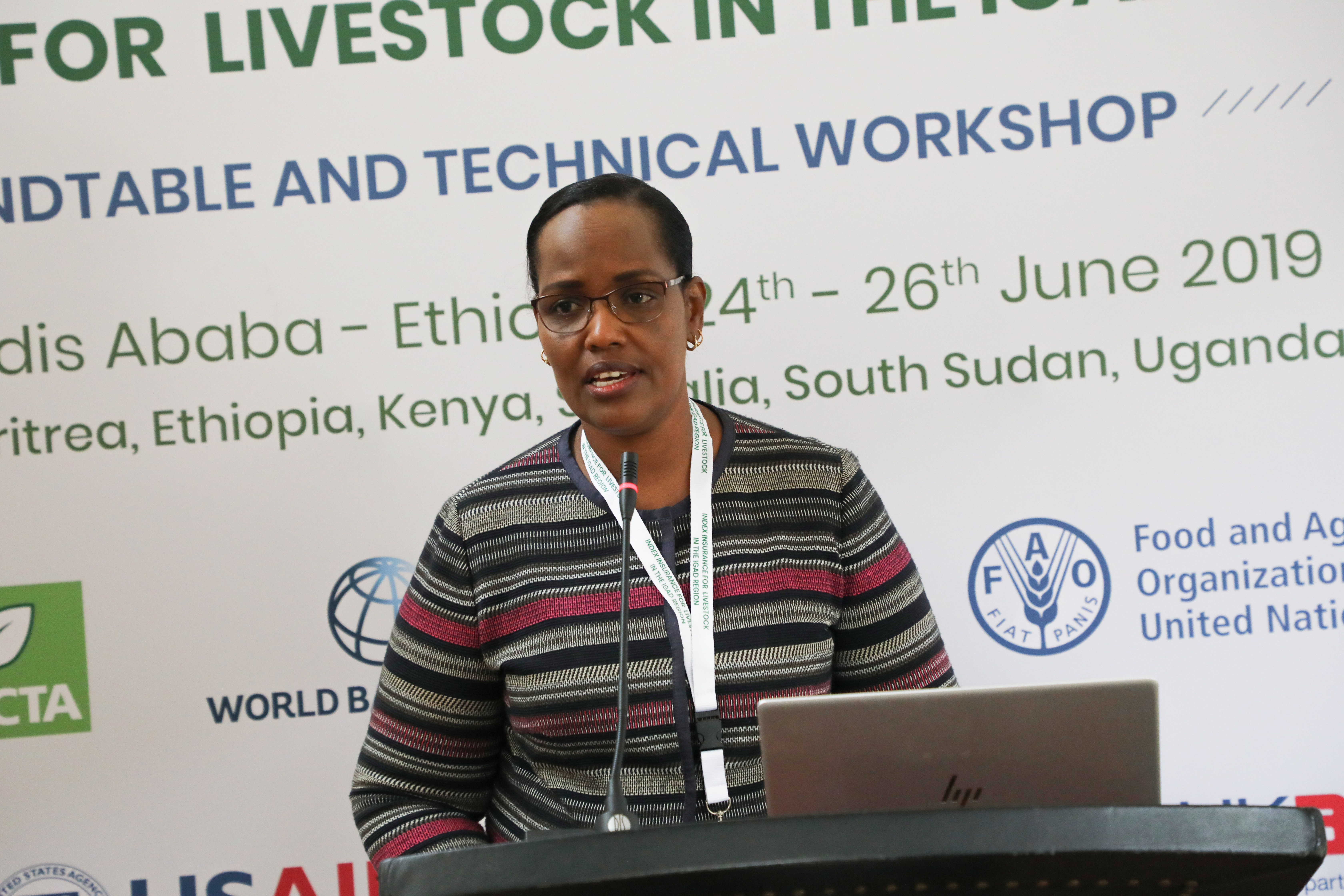The photograph features an African American woman, approximately 45 years old, giving a speech behind a black podium. Her black hair, combed back with a side parting, and black skin are clearly visible. She is wearing glasses and small hoop earrings. Her eyes are brown, and her mouth is slightly open as she speaks into a small attached microphone. She is dressed in a long-sleeve, horizontally striped sweater with red, black, grey, and white colors, and around her neck hangs a white lanyard inscribed with "Index Insurance for Livestock in the IGAD region."

On the podium, an open silver HP laptop is prominently displayed. Behind her is a large banner with partially visible text that reads, "Technical Workshop for Livestock, Ethiopia, June 24-26, 2019," along with the names of several countries: Ethiopia, Kenya, South Sudan, and Uganda.